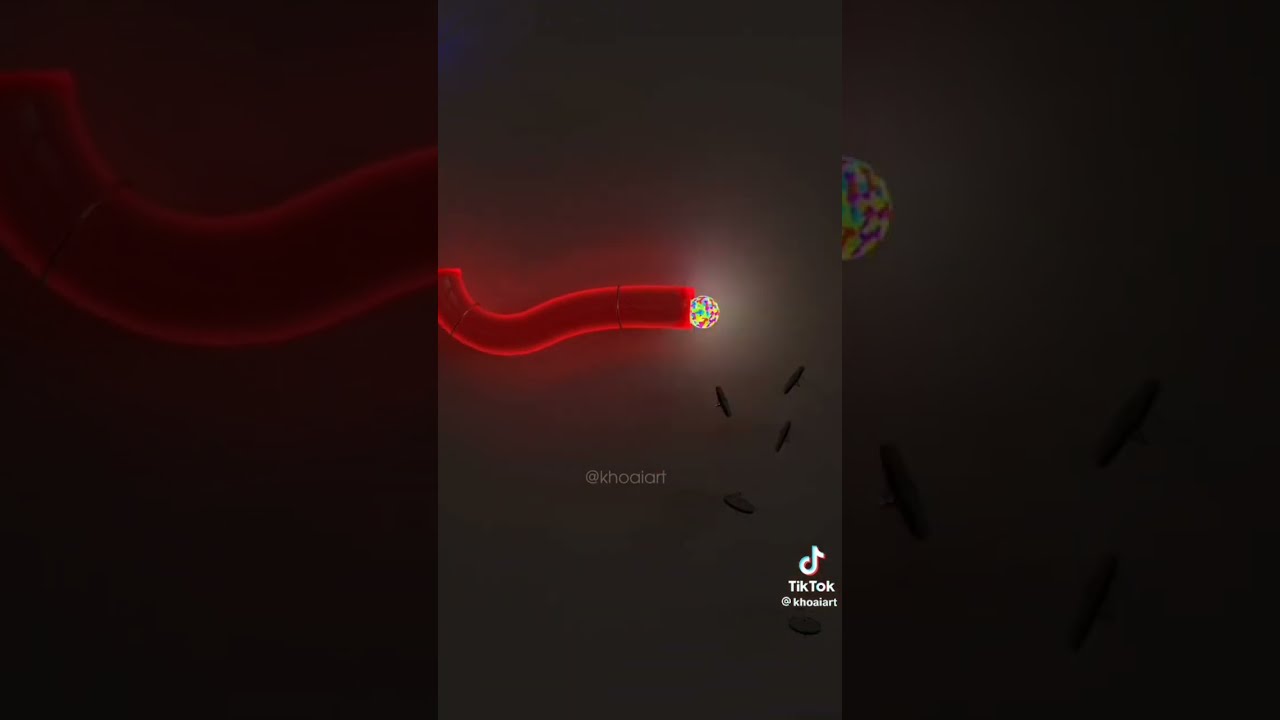This image is a detailed, digitally-generated graphic and appears to be a screenshot of a TikTok video. The TikTok logo and the username "Coalart" are present at the bottom right of the image. The central focus is a luminous, 3D-rendered squiggly figure that resembles a stretched out, glowing red neon tube. The tube is outlined with a neon-like glow and appears to be lit up. Attached to the upper right end of this tube is a small, intricately colored disco ball that shines with multiple bright colors. The entire composition is set against a dark, gray background. The video also displays four indistinct, dark shadows at the bottom, which are difficult to clearly identify but vaguely resemble boats, fish, or even cockroaches. The overall impression is of a neon digital artwork with a mix of vibrant and subdued elements.